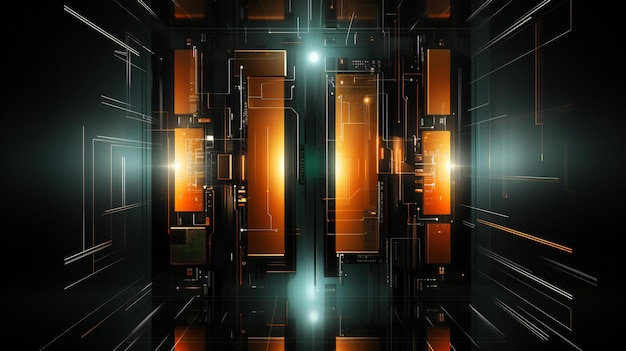This is a detailed, computer-generated graphic depicting a futuristic, dark room with a vault-like atmosphere. The room features slightly cantered black walls on the left and right, adorned with intricate gold and white lines forming circuit board patterns. The shiny black floor reflects a central light source, giving the space a polished and sleek appearance. At the center, the focal wall is composed of orange and gold rectangular panels, divided into four sections resembling a door with windows. These panels emit a medium dark orange glow and are illuminated by bright white lights both at the upper left center and lower bottom center. The overall scene suggests a high-tech environment, with a striking contrast between the dark, reflective surfaces and the glowing light sources.